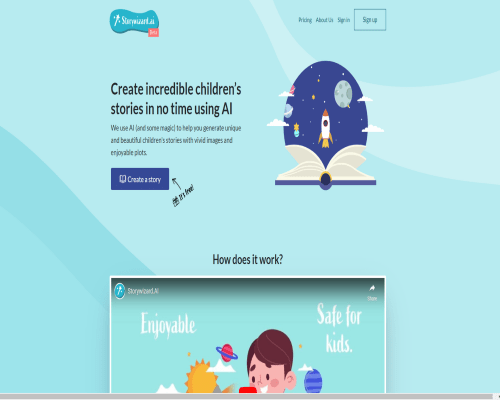A detailed screenshot of a children's educational website displaying its homepage is shown. At the top of the page, there are navigation options including "Pricing," "About Us," "Sign In," and "Sign Up," with "Sign Up" prominently displayed inside a rectangle. The main banner reads, "Create incredible children's stories in no time using AI." This is followed by a subheading that elaborates, "We use AI and some magic to help you generate unique and beautiful children's stories with vivid images and enjoyable plots."

Below this, there is a rectangular button in blue with white text that says, "Create a Story." Next to this button is a small arrow icon for emphasis and what appears to be a hashtag symbol, denoting that it’s free. Additionally, there is a prompt to learn more about the process by clicking on "How does it work?"

An embedded image within the screenshot showcases another computer screen with the words "Enjoyable" and "Safe for Kids" alongside a picture of a smiling boy surrounded by illustrations of planets, emphasizing the imaginative and child-friendly nature of the website.